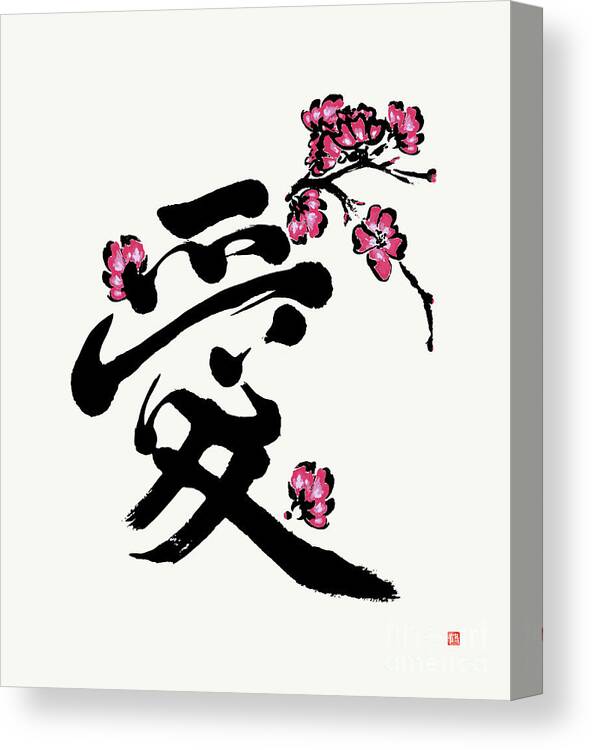This detailed digital painting features a prominent black Japanese calligraphy symbol positioned at the center on a white background. Surrounding the symbol, delicate cherry blossoms with pink petals edged in black and hints of white at their centers are artfully arranged. These flowers extend from the branches, appearing primarily at the upper right, top left, and bottom right areas of the painting, creating a circular flow around the calligraphy. The painting also includes subtle twigs protruding from the blossoms, enriching the intricate details of the floral elements.

The calligraphy symbol itself is complex, containing forms that resemble a swooping line like a skateboard ramp, a mirrored “E” shape, a Nike checkmark, and elements that evoke the image of a racer’s hurdle with a stick beneath it. On the bottom right corner, there is a distinct red and white Japanese character stamp, serving as an artist’s signature or watermark, lending authenticity to the work. Additionally, the painting gives a visual impression of depth due to a slight gray edge on the left side, suggesting a slight tilt or three-dimensional perspective. Overall, this image exemplifies a digital rendition inspired by traditional Japanese canvas art, crafted with precision and cultural symbolism.